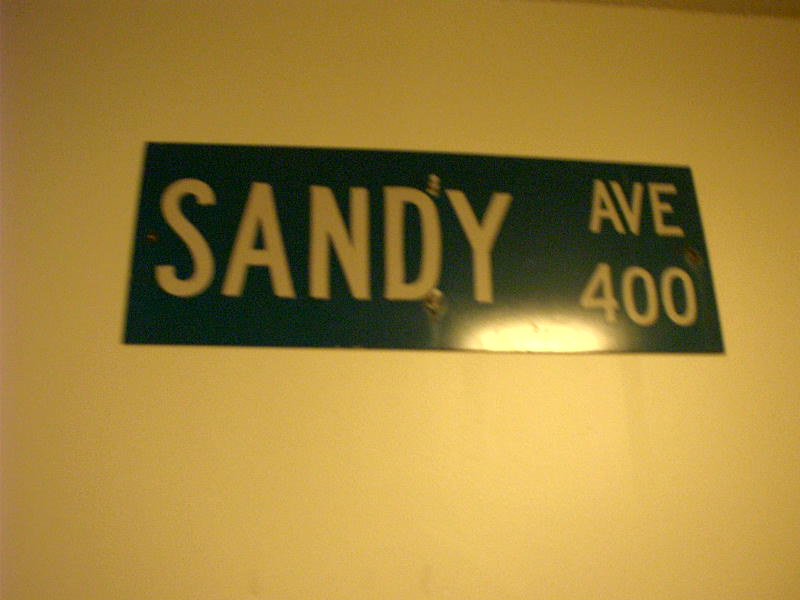This color photograph, taken indoors, depicts a white wall adorned with a green metal street sign reading "Sandy Avenue 400." The rectangular sign is securely fastened to the wall by two central screws, one towards the top and the other towards the bottom. Noteworthy is the interplay of light within the room, which casts a noticeable glare towards the lower right corner of the sign, adding a touch of realism to the image.